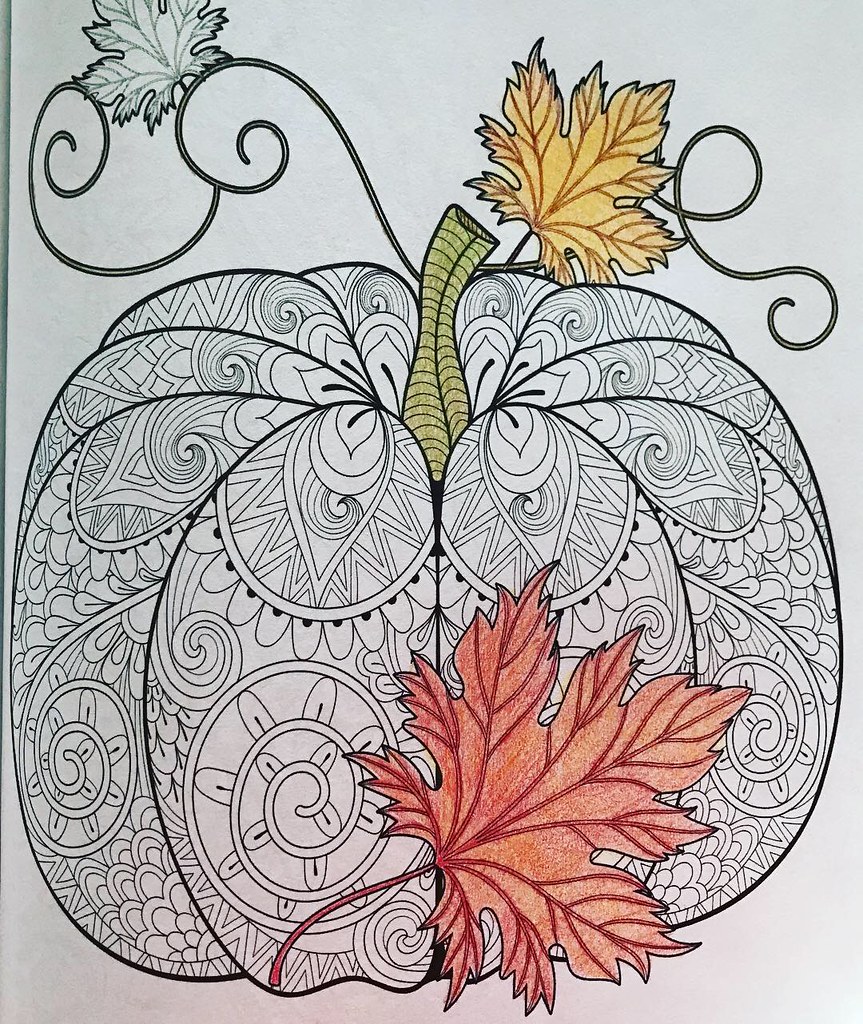This illustration depicts a pumpkin with intricate segments designed for coloring, likely sourced from a coloring book. Most areas remain uncolored, enhancing the contrast with the few vividly painted elements. At the base of the pumpkin, a red leaf is connected, while a green stem emerges from the top, accompanied by a yellow leaf. Additionally, there's another leaf that hasn't been colored yet, all seemingly rooted at the pumpkin's base. The pumpkin's sections feature ornate, floral-like patterns, offering various possibilities for coloring. The entire drawing is set against a plain white background, typical of coloring book pages.